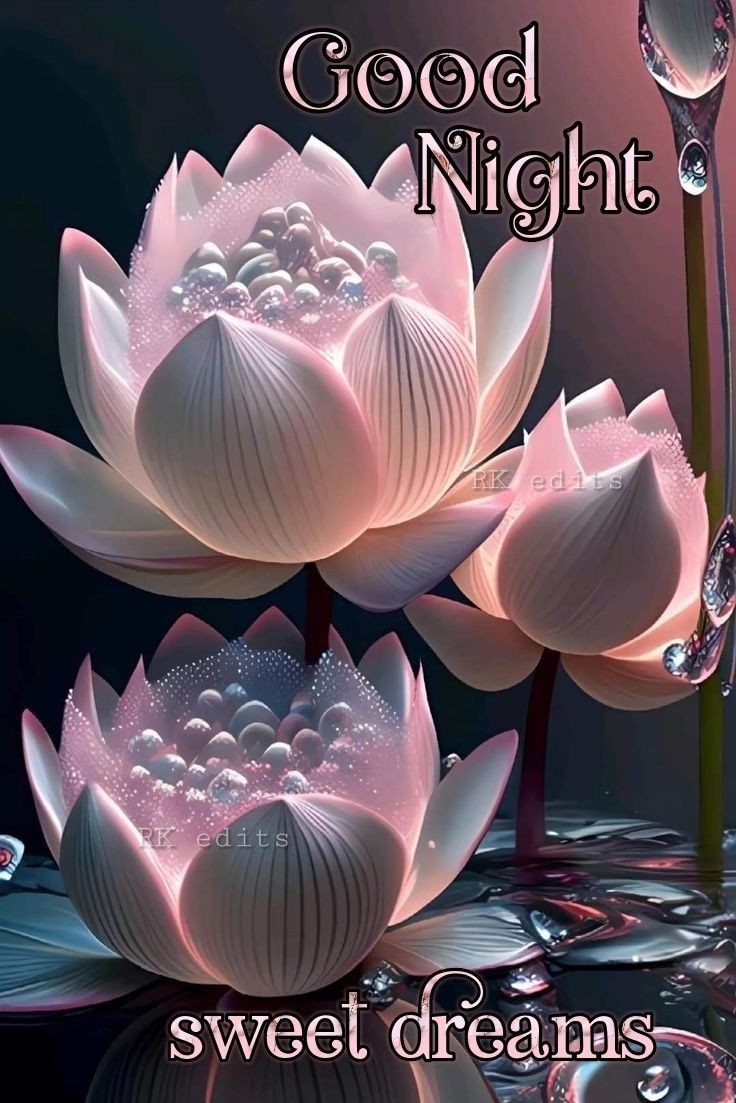The image depicts an artwork designed as a poster or book cover with a striking color scheme of black, burgundy, and dark pink. The caption "Good Night" is prominently displayed at the top in pink letters outlined in black, while "Sweet Dreams" is centered at the bottom in the same style. The centerpiece of the artwork features a collection of glowing pink and white water lilies and lotus leaves. The flowers, some fully open and some still buds, contain small white spheres reminiscent of pearls or soapy bubbles, with a liquid-like appearance. The background transitions from black at the bottom to a dark reddish pink at the top, creating a dramatic, dreamy atmosphere. At the bottom, there are leaves and soapy dots suggesting water droplets on a lake, from which the lotus leaves stem out. A prominent bulb with liquid dripping can be seen on the upper right side of the image, adding to the surreal and serene composition.